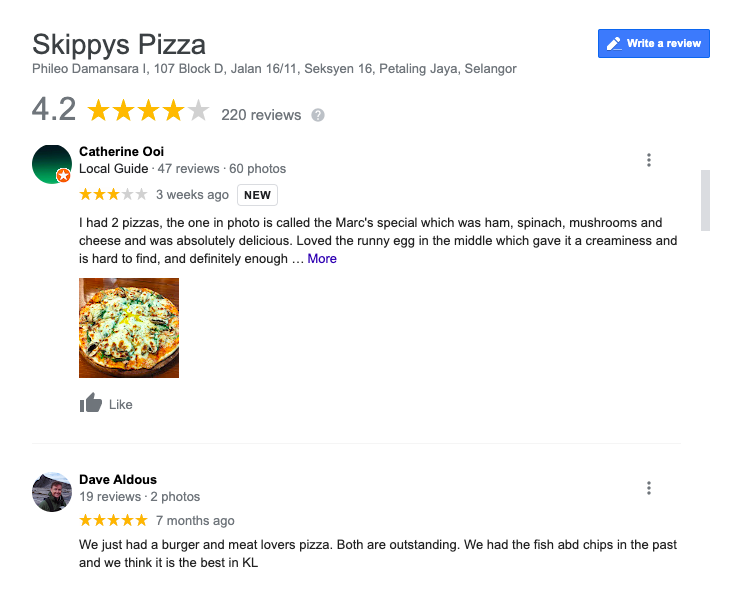On a popular review website, the page for Skippy's Pizza, located at 107 Block D, Jalan, features a detailed layout. On the right-hand side, there's a prominent blue box labeled "Write a Review" along with an edit function. The establishment boasts a rating of 4.2 stars out of 5, as indicated by four gold-colored stars out of five, from 220 reviews. A question mark icon is present next to the rating.

Beneath the rating, there's a green circle icon featuring a star, showing a review from Catherine Oi, a local guide with 47 reviews and 60 photos. Her review, posted three weeks ago, awards Skippy's Pizza three stars. Catherine describes her experience with two pizzas, highlighting the "March Special" pizza in the included photo. This pizza, topped with ham, spinach, mushrooms, cheese, and a runny egg in the middle, is praised for its deliciousness and creaminess. Catherine notes that while the pizza is hard to find, it is definitely sufficient. To read the full review, users must click the "more" link. 

A photo of the thick-crusted "March Special" pizza accompanies the review, and users have the option to like the post. Below Catherine's review, Dave Aldis shares his experience with 19 reviews and two photos. Seven months ago, he rated Skippy's Pizza five stars, commending both the burger and the meatlovers pizza, declaring them outstanding. Dave also mentions having tried the fish and chips previously, which he and his companions consider the best in Kuala Lumpur.